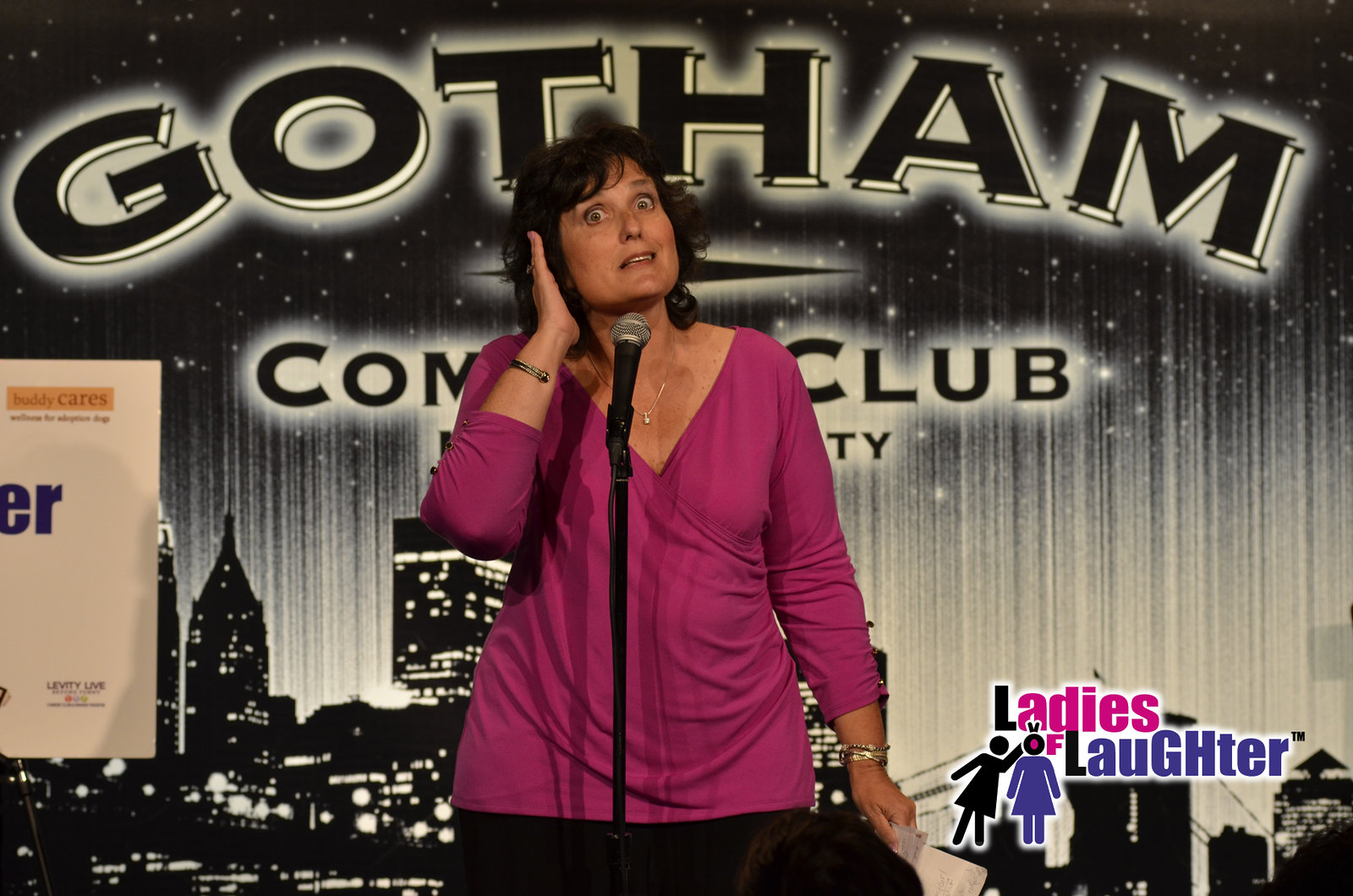A horizontal rectangular photograph serves as an advertisement for Gotham Comedy Club, featuring a middle-aged woman performing on stage. The woman, dressed in a long-sleeved, v-neck top in a vivid shade of pinkish-red or fuchsia and dark bottoms which are mostly out of the frame, stands at a microphone, likely delivering a joke or punchline. Her dark shoulder-length hair frames her expressive face, adorned with surprise. She holds a paper in her left hand, while her right hand, adorned with a bracelet or watch, is raised to her ear. Behind her is a cityscape set against nighttime curtains with the large text "Gotham Comedy Club" partially obscured by her figure. In the lower right corner, emblazoned in black, pink, and purple letters, is the text "Ladies of Laughter," accompanied by two silhouetted female figures - one in black and the other in purple, with the latter forming the 'O' in "of" within the logo. To the side, a blue and white rectangle, possibly a poster, is partially visible.